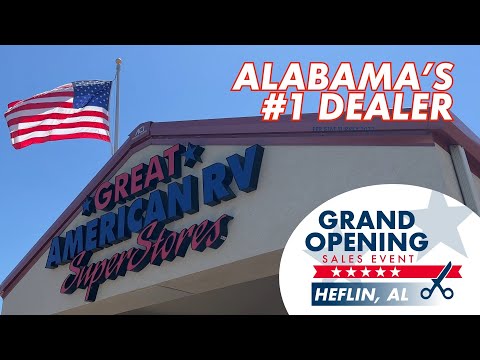This image showcases the top facade of the building for Great American RV Superstores. The building features a light brown roof and tan walls, all captured under shade. Central to the image is the store's sign: "Great American RV Superstores" with 'Great' in red, flanked by blue stars, 'American RV' in blue, and 'Superstores' in italicized red font beneath it. An American flag adorns the left side of the building, illuminated by sunlight. The upper right corner of the image displays the text "Alabama's number one dealer" in white with a red border. A white circle with gray stars occupies the bottom right corner, featuring the words "Grand Opening" in blue letters, "Sales Event" in red letters below, and "Heflin, Alabama" at the bottom. A red ribbon cutting ceremony is depicted in the middle of the image with blue scissors. The photo is framed with black borders at the top and bottom.